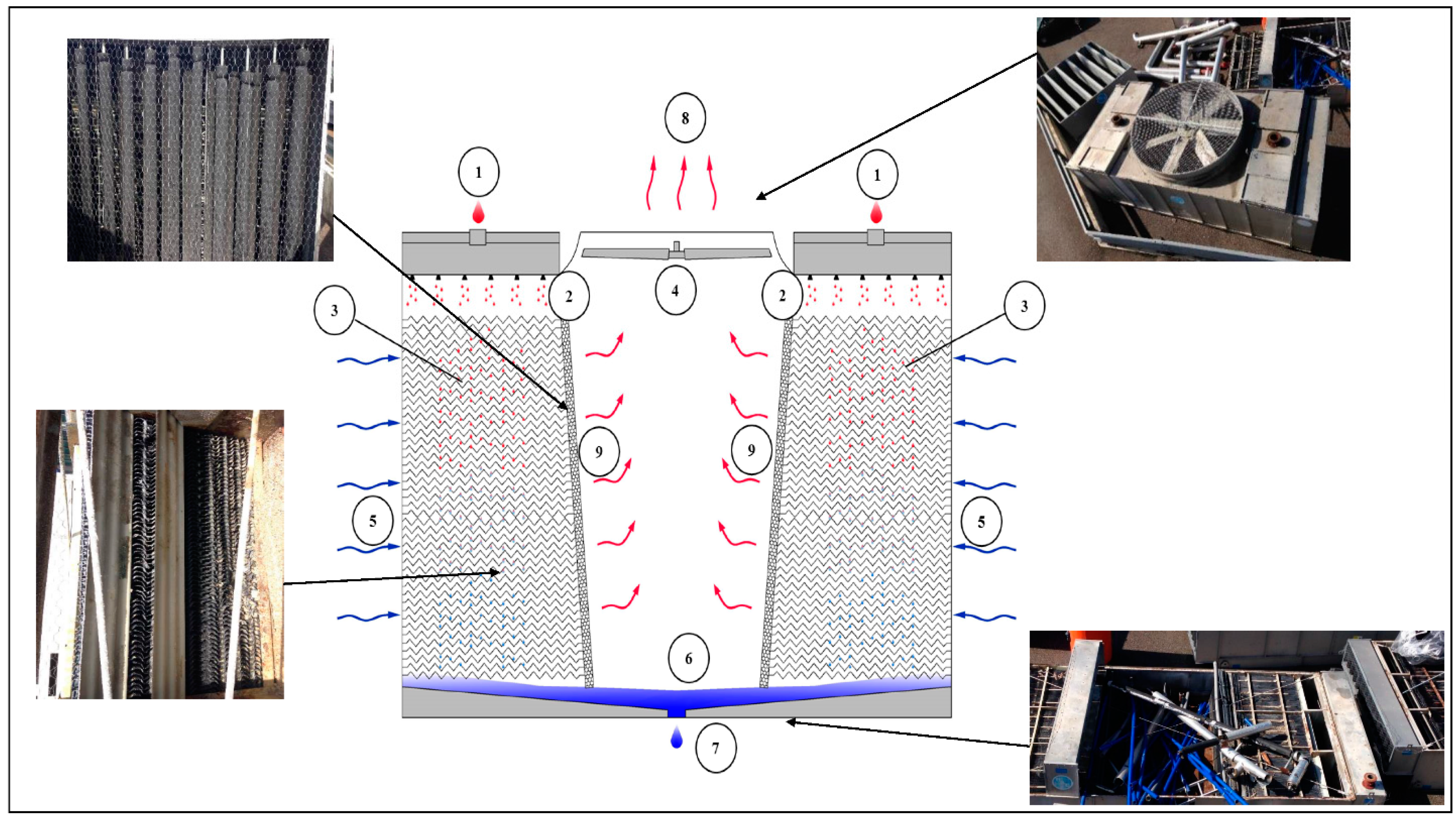This image is a detailed diagram of a heat distribution unit, possibly a furnace or a heating system. At the center, there's a digital illustration resembling a cup, illustrating the process by which heat escapes through vents. Surrounding this central image are additional pictures that depict the assembly and inner workings of the unit. One image focuses on the vented section, which likely houses the fan. Another image appears to show the top of the unit, where a turning mechanism is situated, possibly indicating a component that facilitates air movement. Further images might reveal an internal view of the unit, showcasing various parts including some blue components. A comprehensive diagram highlights the airflow process: cold air enters through the sides, becomes heated, and exits as warm air through the vents. This combination of diagrammatic and photographic elements provides a thorough depiction of both the external and internal mechanisms of the heat distribution unit.